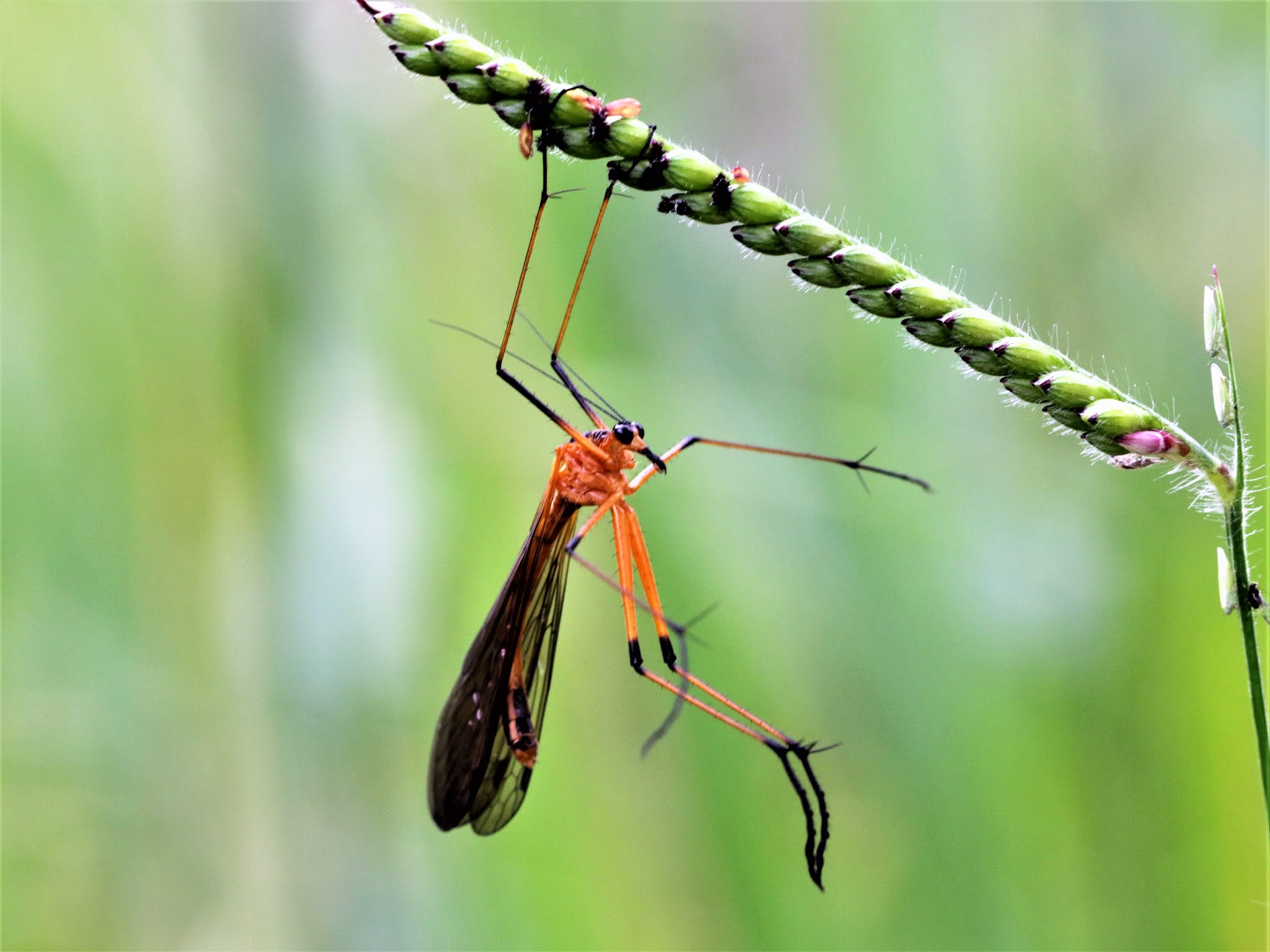The image captures a strange insect with an elongated body and delicate wings, resembling a mosquito but with unique features. The insect's body is a vibrant golden orange color with a distinctly black proboscis and dark eyes. Its legs are a striking combination of orange and black, with hooked ends that grip a slender, green, grass-like plant. The insect hangs by just two of its legs, while the other four dangle beneath it. Its long wings are closed, predominantly black with subtle orange specks, and larger than its body, extending from its thorax and covering its abdomen. The plant it clings to has a green stem lined with tiny, budding pods tipped with purple, suggesting future pink blooms. The antennae of the insect are prominently raised in the air, and the backdrop of the image is a soft, blurred mix of greens and silvers, providing a tranquil, out-of-focus foliage background. The branch stretches from the right side toward the top left, framing the scene and emphasizing the insect's precarious perch.